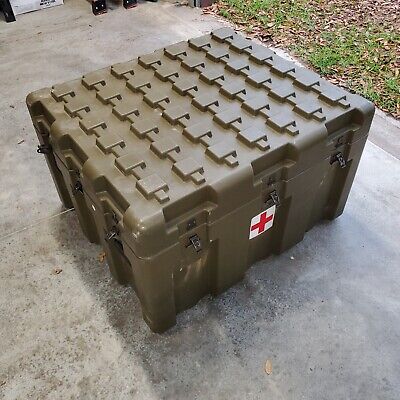The photograph features a large military-style crate made of olive green plastic with a textured, interlocking top surface. The crate, intended for stacking, is adorned with a prominent first aid sticker—a white square with a red cross. The crate is closed and features three black latches on each visible side, though some are unlatched. Positioned on a concrete surface, the image captures details of the setting, including green grass and brownish leaves in the top right corner. The photograph appears to have been taken outside on a partly cloudy day, emphasizing the outdoor environment of the scene.